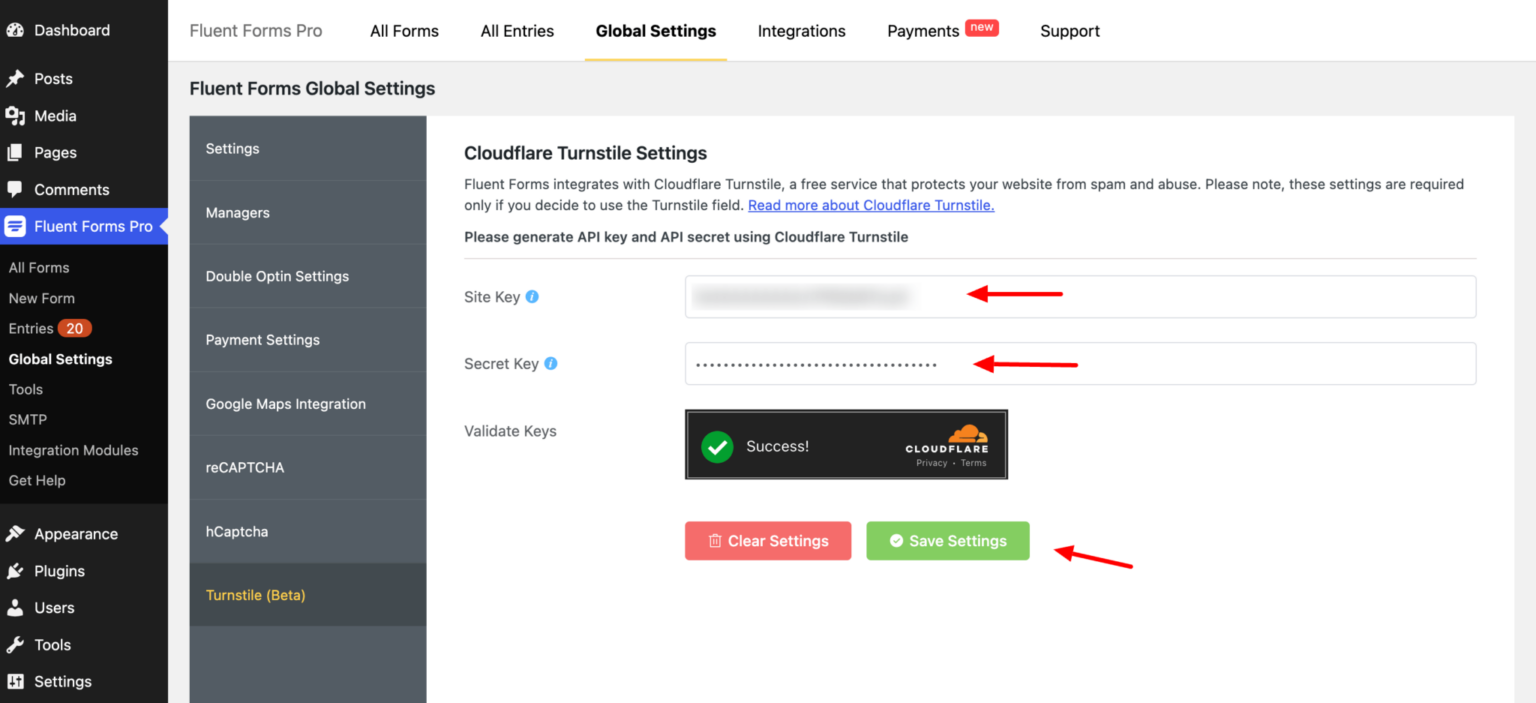The image captures a screen from an online application with an off-white background. On the left, there are two vertical frames: the first one is black, and the adjacent frame has a grey background. The central portion of the image displays a series of rectangular buttons accompanied by red arrows pointing towards them. At the top of the section with the buttons and arrows, there is a heading in dark grey text that reads "Cloudflare Thumb Style Settings." Below this heading, in smaller grey text, it states, "Fluent Forms Integrate Cloudflare Thumb Style, a free service that protects your website from spam and abuse. Please note these settings are required."